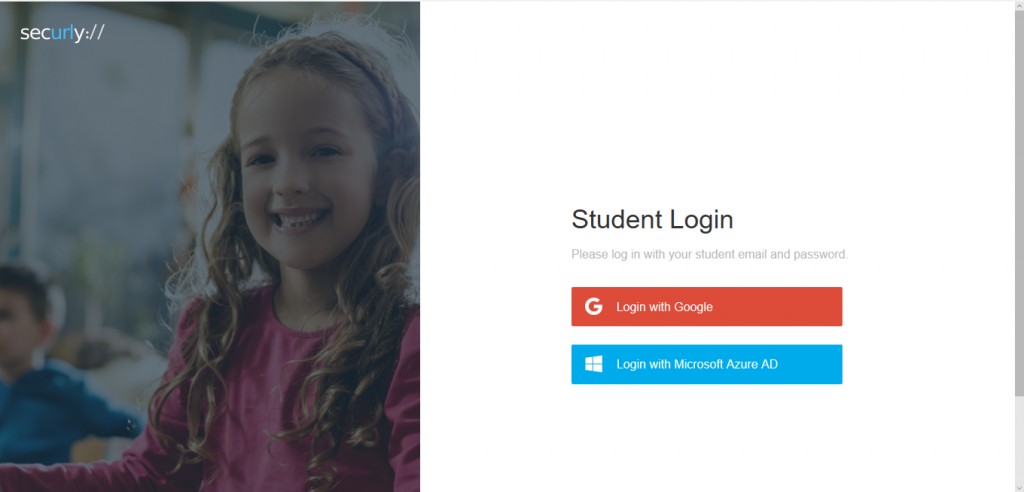The image is a screen capture of an online application interface with a white background. Located at the upper left side of the screen, there is a photograph of a young girl wearing a long-sleeved pink top. She has long, curly brown hair and is smiling. Next to her, on her left side, is a small blue icon resembling a boy, also colored in blue. At the upper left corner of the screen, written in a combination of white and blue texts, is the phrase "securely://".

To the right of the image, still on the white background, appears the blue text "Student Login". Beneath this text, a smaller, light gray text instructs, "Please login with your student email and password." Below these instructions, there is a prominent red rectangular button labeled "G Login with Google" in white text. Underneath the red button, there is a blue button with white text that reads "Login with Microsoft Azure AD."